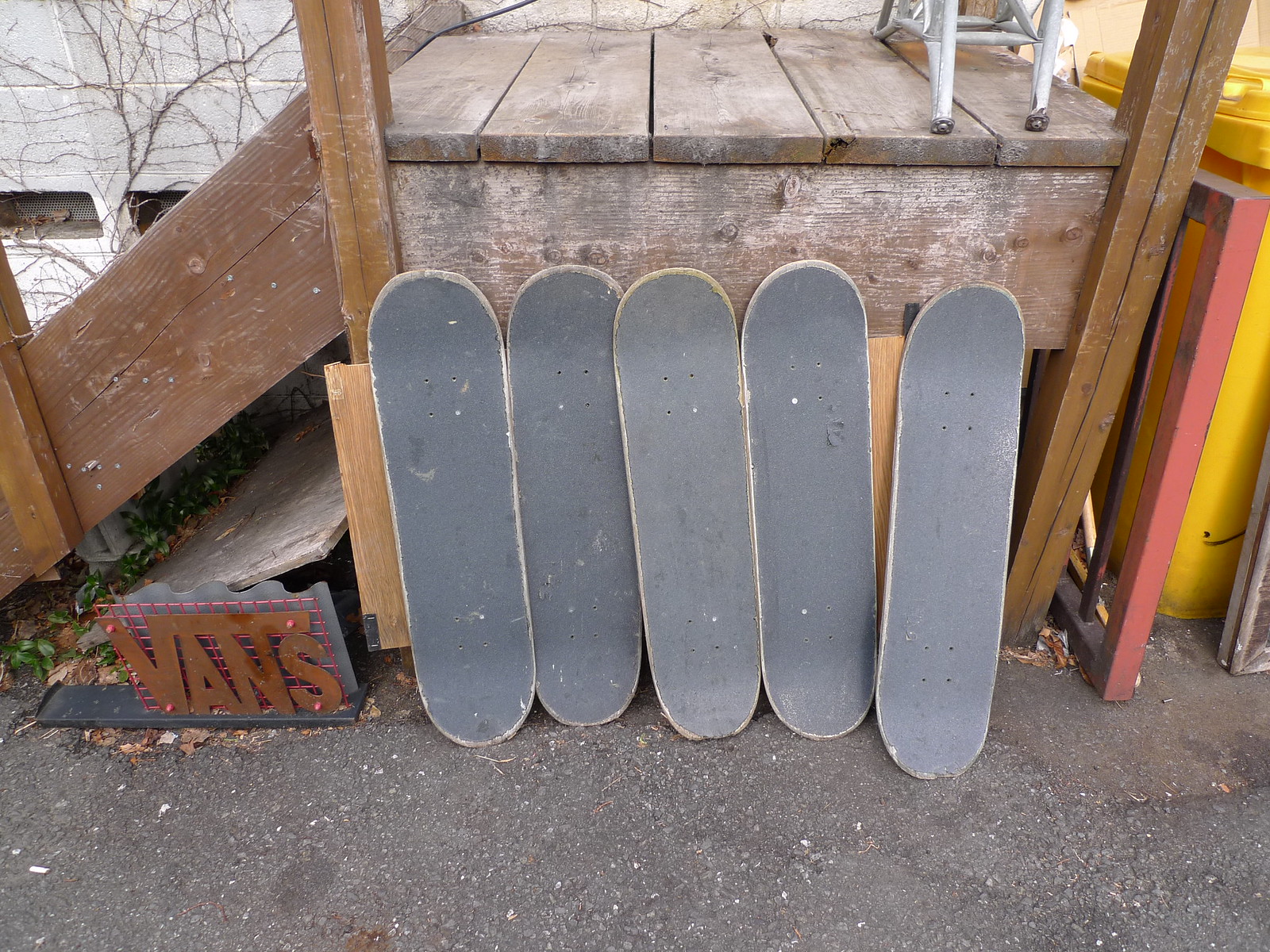The photograph appears to be a candid shot taken with a personal device, capturing a scene of five gray, wheel-less skateboards lined up against an aged, brown wooden deck that features white paint. The deck, possibly part of a porch, leads up via a short set of stairs, and the sidewalk they rest on is tarmac. To the left of the skateboards lies a small 3D outline block bearing the "VANS" logo. There is a bare tree in the background suggestive of winter, and a yellow trash or recycling bin positioned on the right near the white, vine-covered walls of a house. The overall ambiance is rustic with a juxtaposition of casual outdoor elements, giving it a homely yet somewhat worn look.